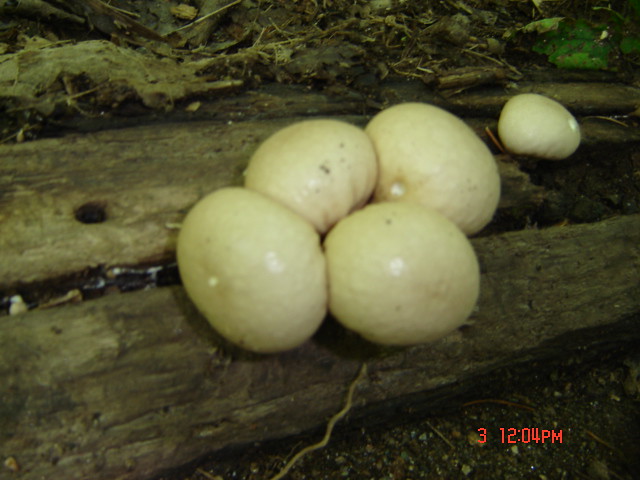The photograph captures a damp, woody area featuring an arrangement of five creamy, off-white puff-like fungi known as Psilocybe weraroa, growing between two heavily weathered, mossy logs. Four of these rounded fungi are clustered closely together, their surfaces appearing glossy and slightly textured, while a smaller one sits in the background to the right. These fungal growths resemble small onions or eggs in shape and size, with some having subtle black dots and a distinct indentation on the one in the back. The setting includes dark soil, rotting leaves, and a small patch of green foliage, hinting at its moist and shaded environment. The photo contains red text in the lower right corner displaying the number "3" followed by "12:04 p.m." The overall scene is slightly out of focus, enhancing the mysterious and earthy ambience.